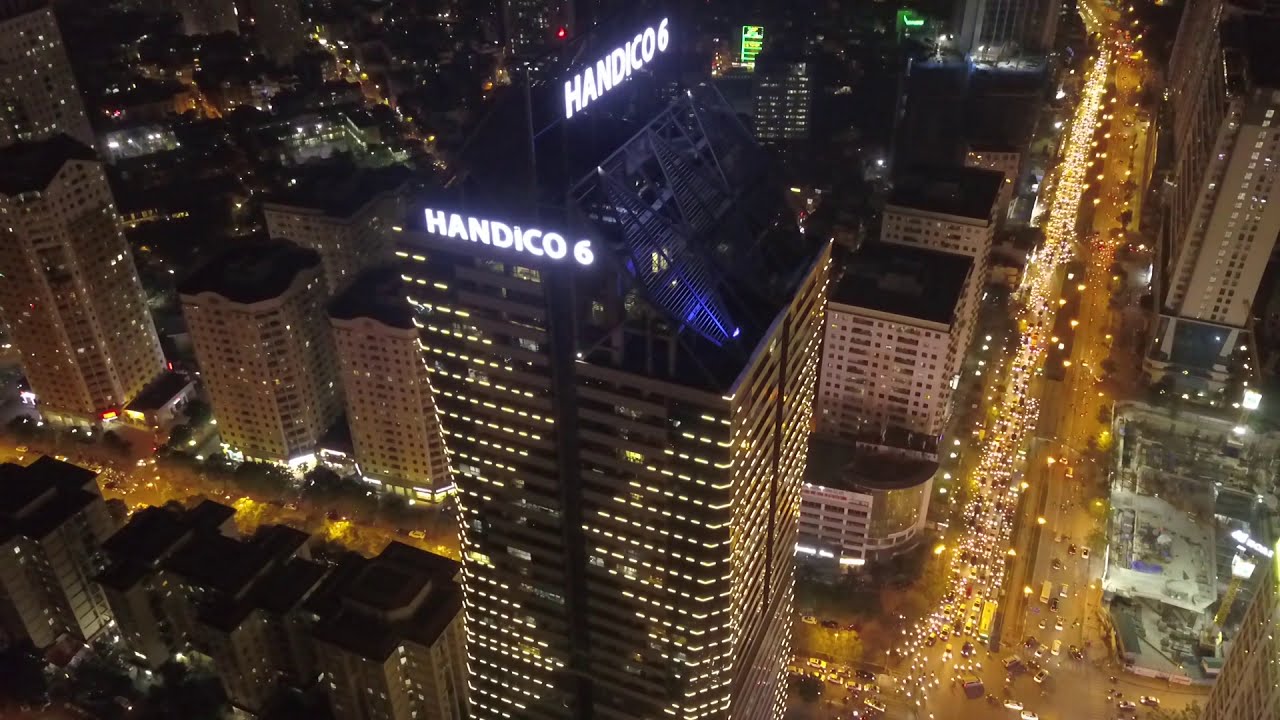This aerial nighttime view of a vibrant city showcases a bustling urban landscape dominated by the prominent Handico 6 building, which stands illuminated at the center of the photograph. The Handico 6, the tallest structure visible, features a dazzling white light display on its top and sides, which reads "Handico 6." This distinctive building also boasts a striking design accentuated by lights along its structure. Surrounding the Handico 6 are numerous multi-storey buildings, some significantly smaller and one particularly glossy, possibly a shopping mall. The streets below are alive with traffic, where the headlights of vehicles create long strips of white and yellow light, adding to the city's dynamic atmosphere. The clarity of the image allows for detailed observation of the buildings and the well-lit streets, emphasizing the lively yet orderly congestion of city life at night. The overall scene is a stunning portrayal of metropolitan grandeur and nocturnal energy.